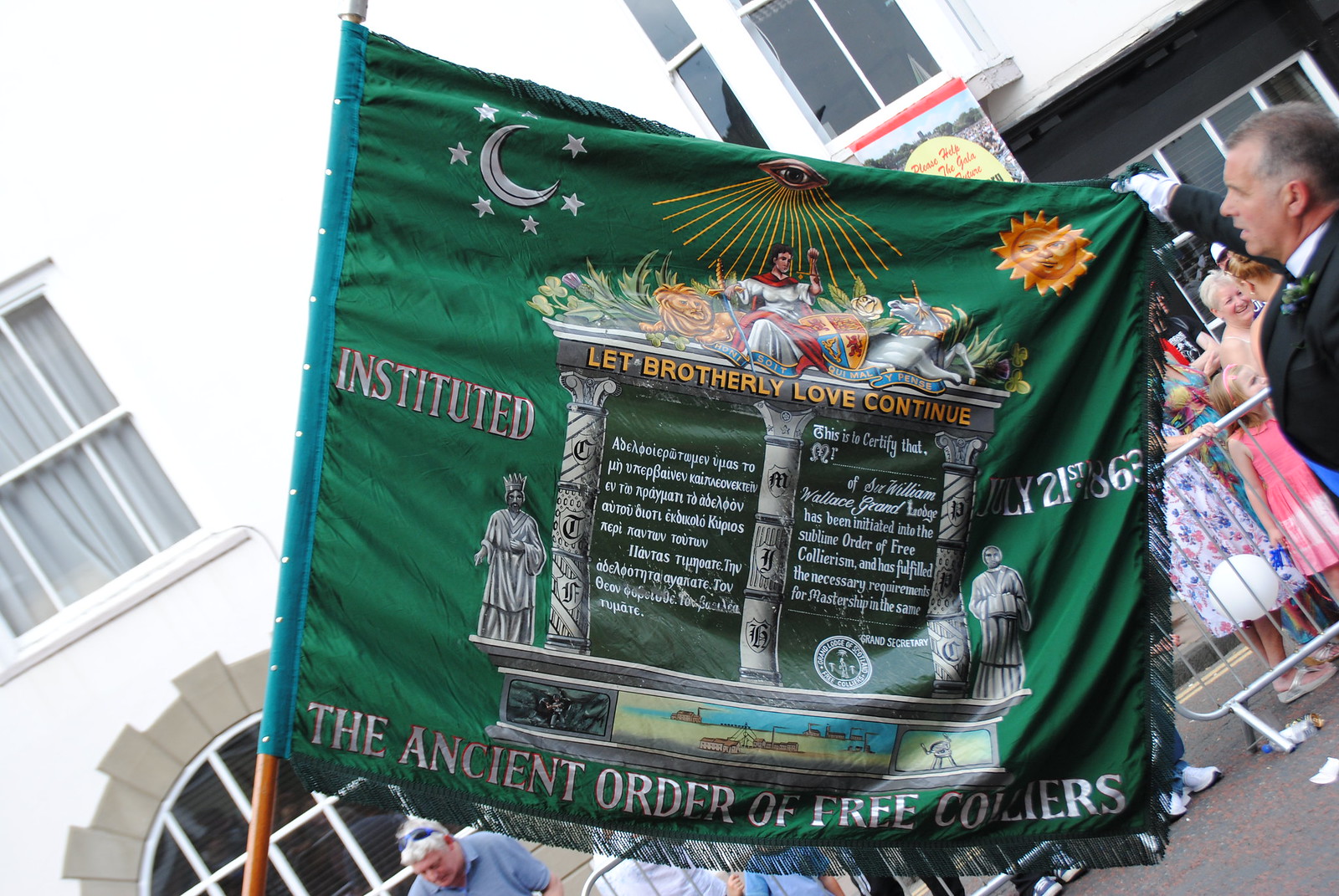In this vibrant outdoor street scene, a crowd stands behind a metal guardrail in front of a white building. Dominating the right side of the image is a man dressed in a black suit with a white shirt and white gloves, holding up a green flag on a brown pole with his right hand. The flag, emblazoned with intricate symbols and text, features a moon surrounded by stars in the top left corner and an orange sun with a face in the top right corner. At the center of the flag, an altar illustration includes an eye at the top, emitting rays downwards. Below the altar, the words "Let Brotherly Love Continue" can be read clearly, with "Instituted" to the left. Further down, partially obscured, the fabric appears to say "The Ancient Order of Free..." The scene is well-lit, indicating it’s taken during a bright day, adding clarity and vividness to the image.